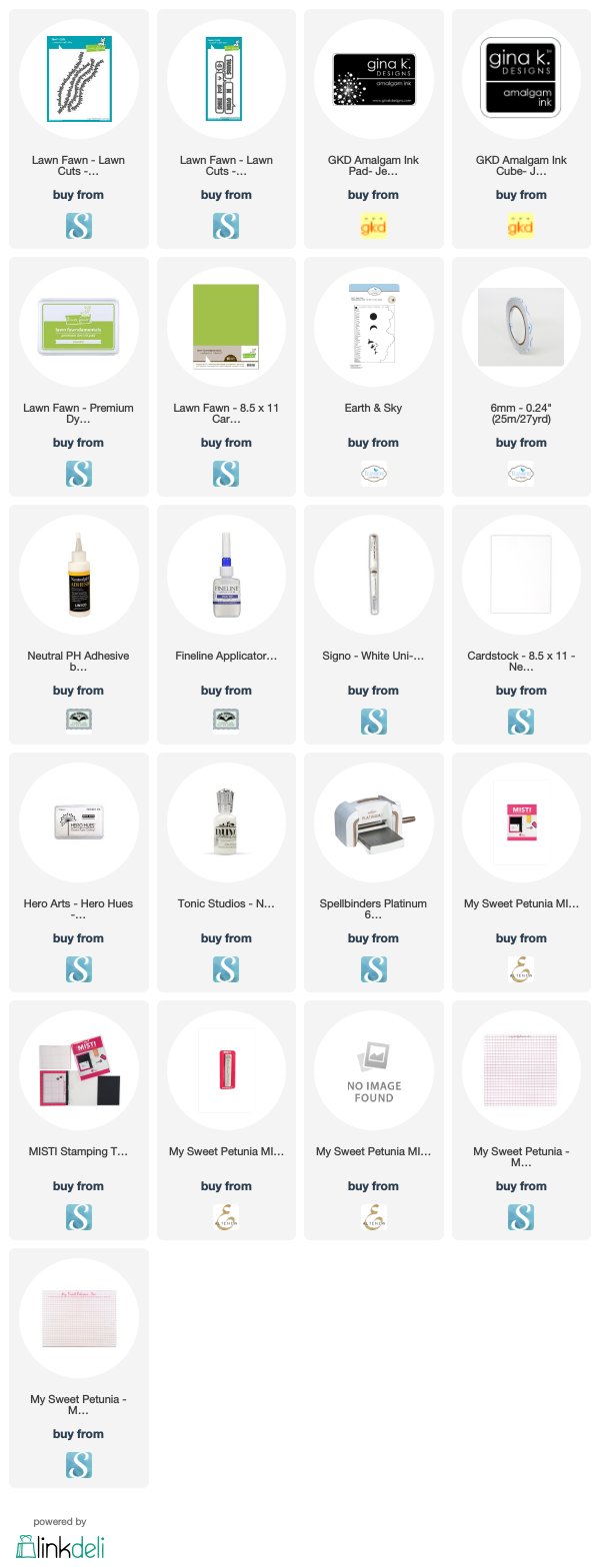In the upper left corner of the image, there is a small square containing an image of wires, accompanied by very small black text on a gray background. Below this, a square encloses the letter "S," followed by another square that seems to depict either the front of a credit card or a black box with some text. The second row consists of what appear to be credit cards or green boxes, each with a small, hard-to-read text beneath them. Moving to the right, there is a small silver ring or earring, accompanied by an illegible price tag. The subsequent row features a variety of items, including what looks like a bottle of water and a mascara tube. The next row displays more varied items, such as a toaster oven with its tray pulled out. Finally, the last row contains various items within each block, including simple colored squares—a red square in one block and a blue square with the letter "S" in another. At the very bottom, the word "link" appears in black text, followed by the word "DELI" in blue text, with each letter separated by hyphens.